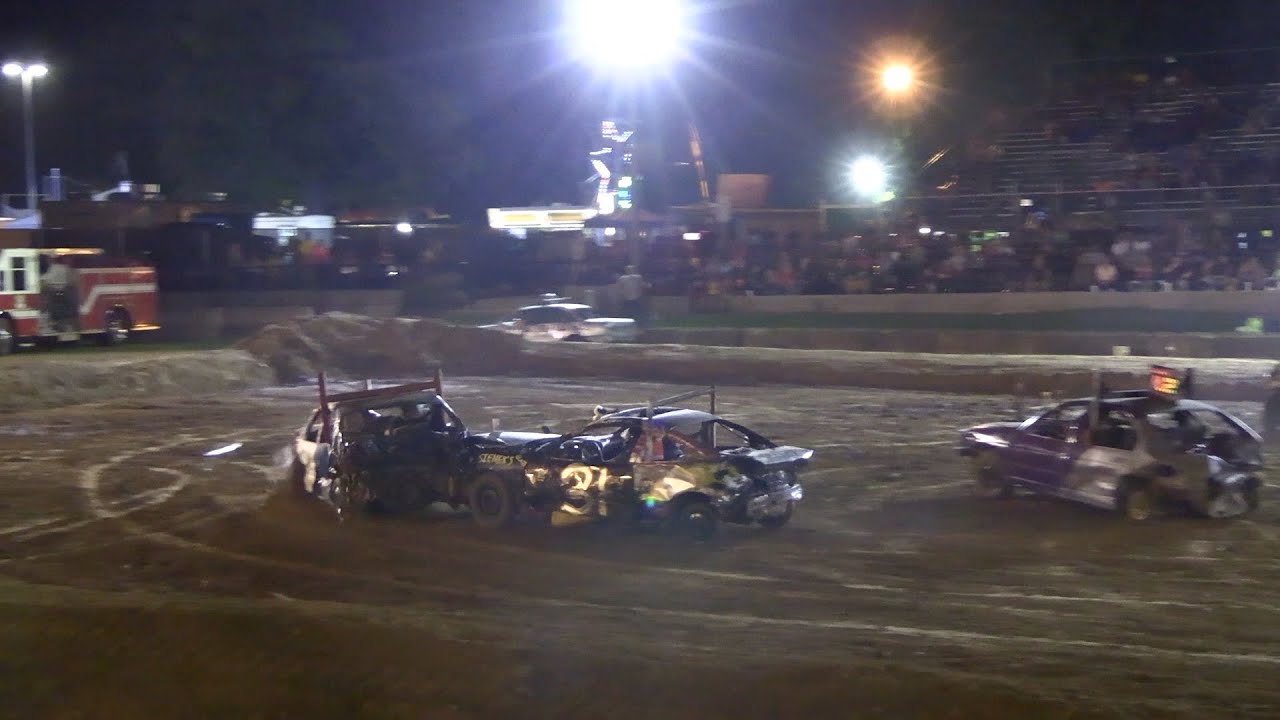The image captures a high-energy nighttime demolition derby, showcasing three heavily damaged vehicles on a dirt track, surrounded by dunes. The cars, which are mid-collision and blurred due to their speed, are banged up, missing windows, doors, bumpers, and feature mismatched, spray-painted components. Each car bears identifying numbers, with the car on the right displaying a prominent "12" and the center car possibly sporting a "31." The scene is illuminated by bright stadium lights, casting a harsh glow on the destructive spectacle. In the background, a large crowd sits in metal bleachers, their details obscured by the darkness and lighting. To the left, a fire truck stands ready, a precautionary measure given the violent crashes. The audience's faint figures and the chaotic motion of the derby cars emphasize the thrilling and perilous nature of the event.